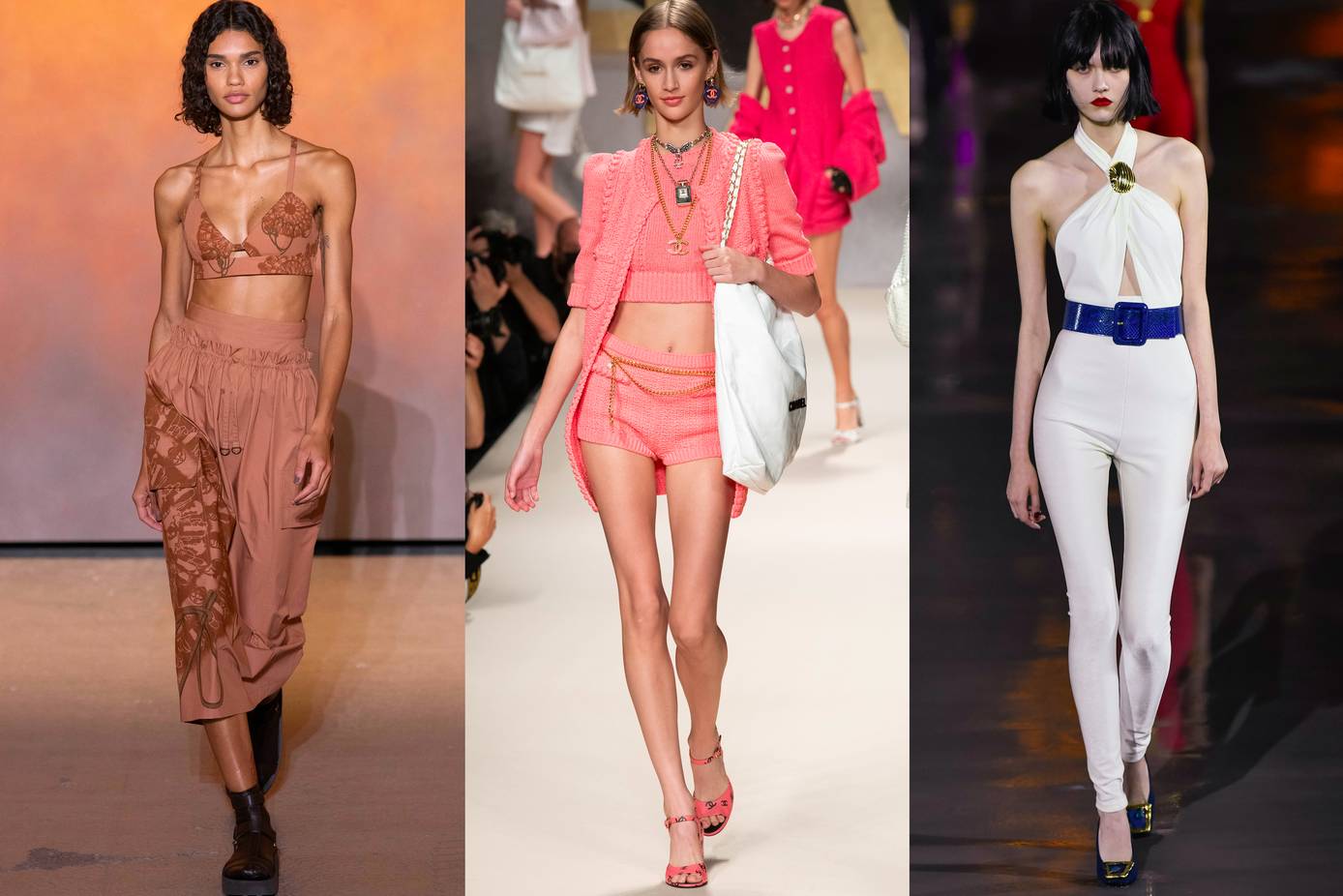The composite image features three runway photographs side-by-side, showcasing models in various high-fashion outfits with a serious expression and similar walking styles as they approach the camera. On the left, an African American woman stands confidently in a beige bikini-style top paired with a beige skirt and black boots. The plain, neutral backdrop contrasts with what looks to be a brown floor. The middle image captures a Caucasian female with short black hair. She sports a coordinated pink ensemble consisting of a crop top, an extended jacket, shorts, and matching sandals. She holds a white handbag in her left hand. There is another female figure partially visible in the background wearing a pink dress, hinting at a bustling fashion show environment. On the right, we see another Caucasian woman, this time with dark black hair, dressed in a white halter top and white pants, accessorized with a blue belt. The backdrop here is understated and out of focus, composed mostly of dark hues, emphasizing the model and her striking outfit.